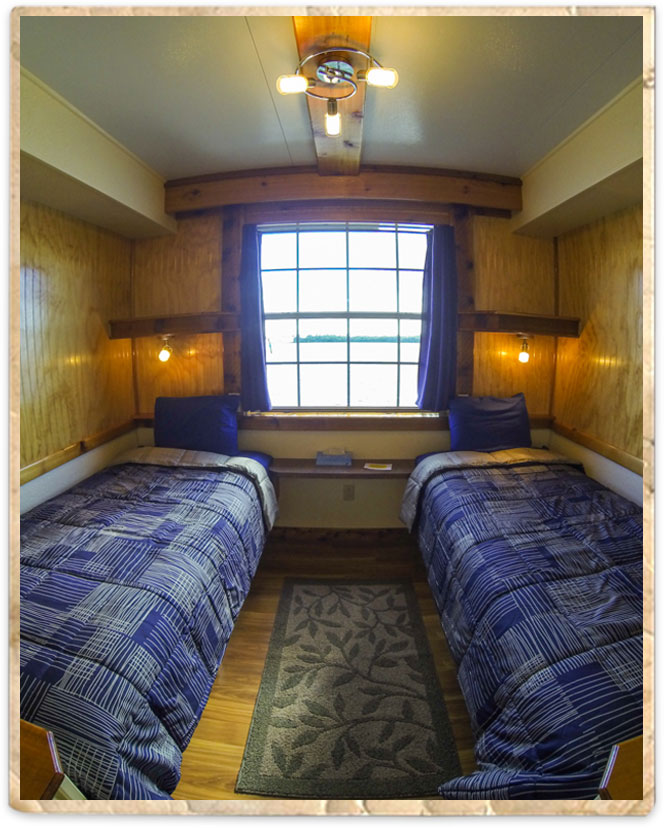The photograph depicts a cozy, symmetrical bedroom, likely situated in a cabin or dormitory, defined by its rustic yet organized design. The room features wooden panels on the left and right walls, seamlessly blending into the brown wooden floor beneath. At the back, a large square window, divided into 16 small squares by its metal frame, offers a picturesque view of a snowy landscape outside. Blue curtains frame the window, complementing the room's color scheme.

Beneath the window, two identical single beds are positioned symmetrically on either side of a central aisle. Each bed is adorned with a blue pillow and a checkered blue and white blanket. A connecting head shelf spans the head of both beds, doubling as both a headrest and additional storage. Above these shelves, small lights illuminate the space, enhancing the room's warm ambiance.

The ceiling, painted a mustard green, features three white lights hanging symmetrically, reinforcing the room's balanced aesthetic. A narrow carpet with a plant theme lies between the beds, adding a touch of nature to the cozy interior. Despite its compact size, the room is well-organized, with every element reflecting a meticulous attention to symmetry and detail.